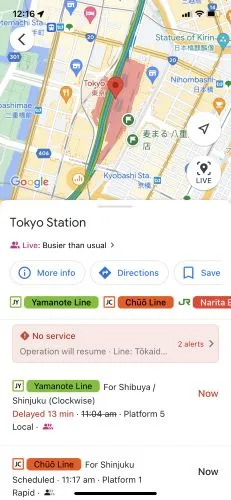A screenshot of a mobile device displays a detailed city map of Tokyo at the top, showing a network of streets and various symbols. The interface includes a back arrow button in the top-left corner and navigation options in the bottom right, such as a small circular icon labeled "Live." Below the map, "Tokyo Station" is prominently featured, along with a purple icon indicating "Live - busier than usual."

Further down, rectangular buttons provide additional options for information, directions, and saving. Various train lines, represented with colored labels and Japanese text, are listed beneath this section. Notably, some services, such as a line highlighted in a large pink box, are marked with alerts like "No service." Other lines, including the Yamanote Line for Shibuya and the Chu Line for Shinjuku, are also mentioned and likely offer more details upon selection. The lower half of the screen is dedicated to these train lines, while the upper half is dominated by the map.